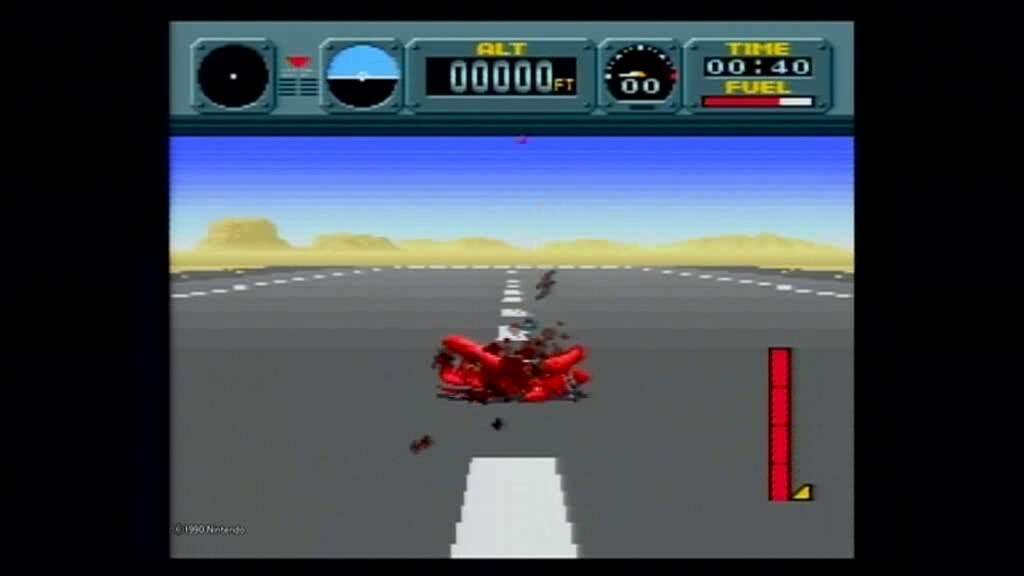This screenshot appears to be from a vintage Nintendo video game, likely from the 1990s, given the observed copyright mark "© 1990 Nintendo." The image quality is low resolution, with pixelated graphics typical of older games. The game seems to be running on an emulator, as suggested by the 4:3 aspect ratio positioned within a widescreen frame, bordered by thick vertical black bars and thinner horizontal bars.

The scene depicts a crash site on an airport runway surrounded by grayish desert mountains. A red, destroyed biplane lies smoking on the runway, which features prominent white dash lines. The control panel at the top of the screen shows various gauges: an altitude indicator displaying "00000 FT," a time gauge reading "00:40," and a fuel gauge partially filled with a red bar. Additional details include maroon debris scattered from the crashed plane, and on the right-hand side, a red bar and a yellow triangle indicator.

Overall, the intricate elements from the control panel and the crashed plane give the impression of a flight simulation game, emphasizing the site's desolation and the detail-oriented interface characteristic of Nintendo's early gaming era.